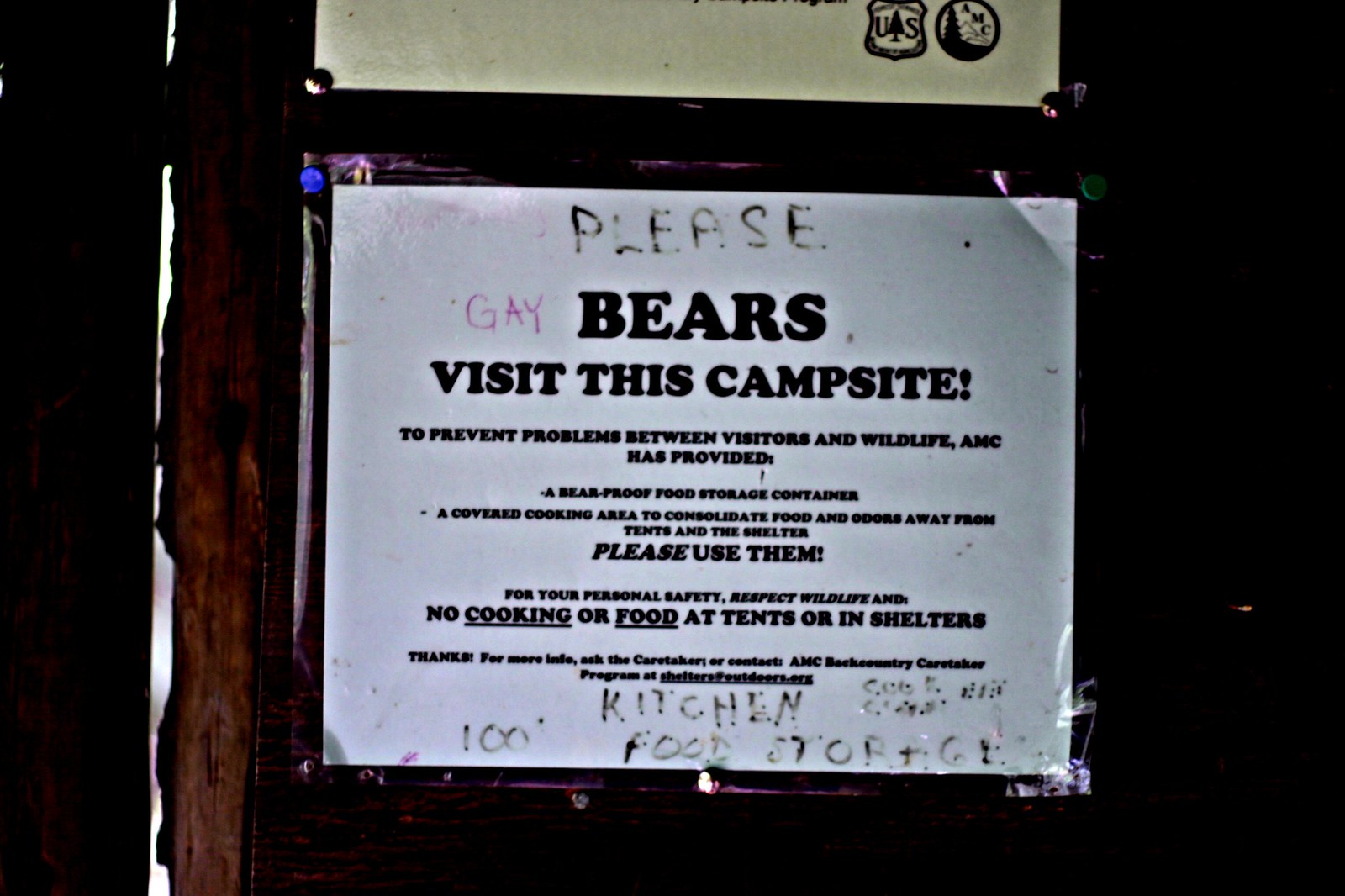This is a nighttime photo of a white warning sign attached to a wooden board at a campsite. The sign, illuminated faintly from a light source coming through a crack on the left side, issues a detailed warning about the presence of bears. It informs campers that to prevent problems between visitors and wildlife, the AMC has provided a bear-proof food storage container and a covered cooking area to consolidate food and odors away from the tents and shelter. The sign emphasizes the importance of using these facilities for personal safety and respecting wildlife by not cooking or storing food in tents or shelters. The words "bears" and "visit this campsite" are prominently displayed. The sign has been defaced with graffiti, including a notable alteration to "please gay bears visit this campsite" and additional, less legible graffiti at the bottom. The background is very dark, indicating that the picture was likely taken late at night.